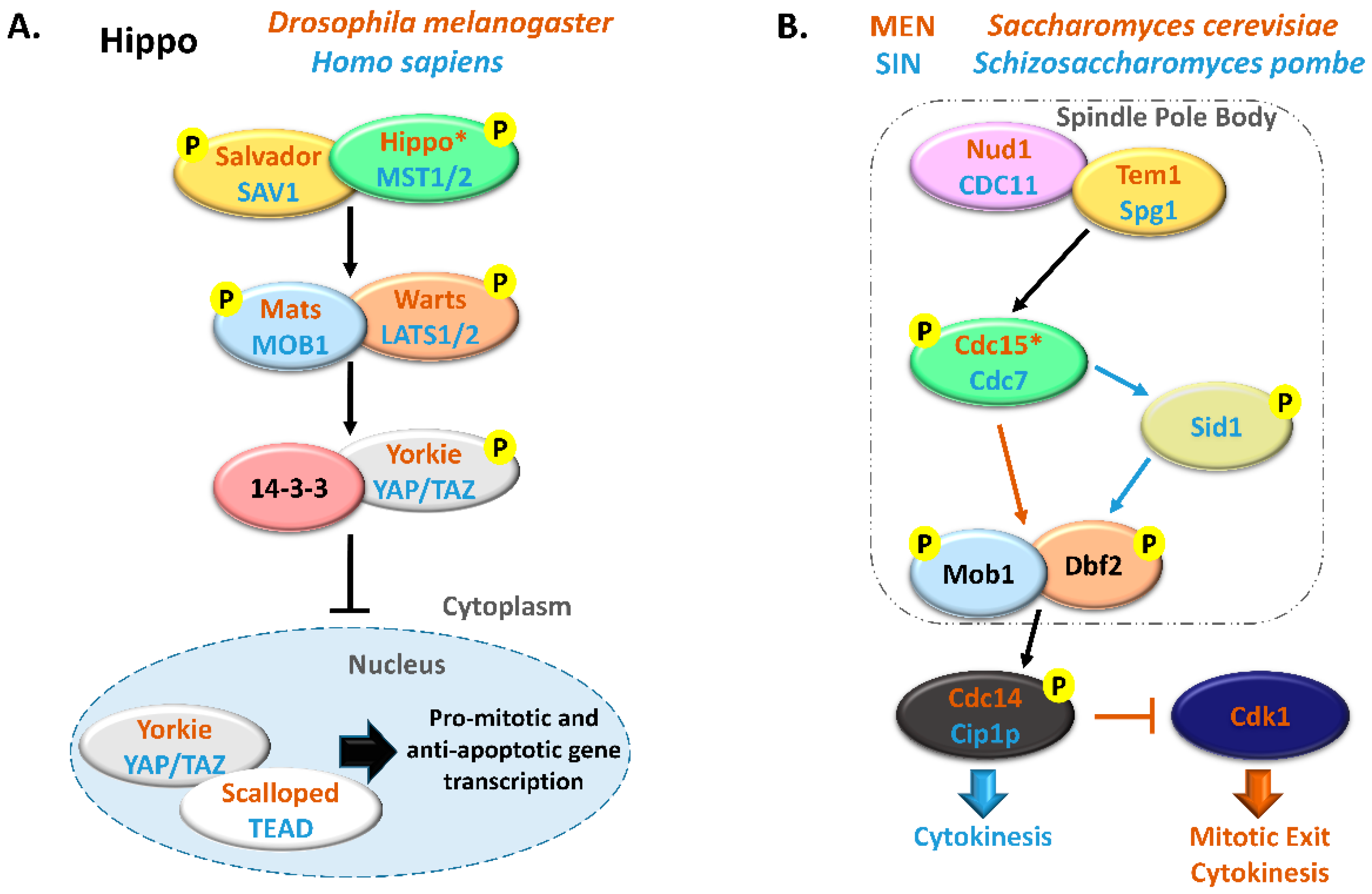The image features a detailed flowchart of scientific information. In the top left corner, there is a black label "A." followed by the word "HIPPO." To its right, in orange text, it reads "Drosophila melanogaster," and directly below this in blue text is "Homo sapiens." Below these labels, there is a yellow oval longer on the left and right sides, labeled "Salvador" in orange text and "SAV1" in blue text. Adjacent to this on the right is a green oval labeled "HIPPO*" in orange text, with "MST1/2" written in blue text beneath it. The green oval also has a black arrow pointing downward, indicating a direction in the process.

Additionally, there are multiple ovals with names inside them, arranged side by side at the bottom, some of which include the word "NUCLEUS" with light dotted blue lines surrounding it. To the far right, there is more scientific data mentioning "Saccharomyces cerevisiae" along with other names and several more ovals leading downwards, suggesting a continuation of a biological or chemical process.